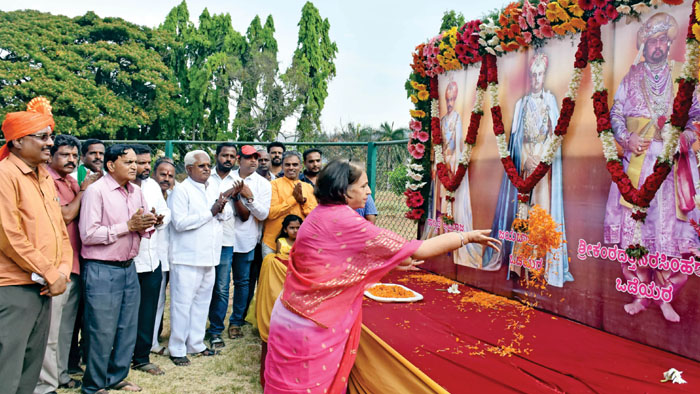The image captures a ceremonial scene likely in India, featuring a gathering of people primarily of Indian descent, standing to the left and extending towards the center and back of the image. They face a richly decorated structure adorned with flowers along the top and sides, vibrant in hues of red and gold. Central to the scene is a woman dressed in a striking red or pink sari, her right arm outstretched as she scatters orange petals onto a large, red-clothed table in front of her. The table is layered with a gold cloth beneath the red one. Behind this table, a mural showcases three religious figures side-by-side, each robed in luxurious attire. The background reveals a chain-link fence with trees bearing green leaves, set against a light blue sky.